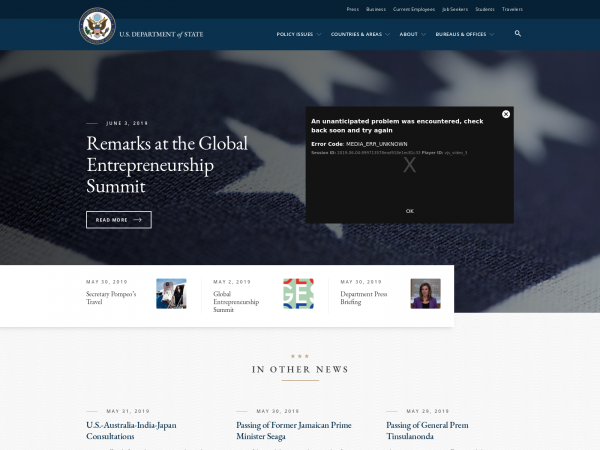In this image, we see a website belonging to the United States Department of State. In the top left corner, the department's name is prominently displayed. To the right, there are several drop-down menus labeled "Policy Issues," "Countries and Areas," "About," and "Bureaus and Offices." A search button is located further to the right.

The main content of the page features multiple sections with headlines and text. One section contains a headline about the Global Entrepreneurship Summit, with a prompt to "Read more." However, it appears there was an issue displaying some content, as an error message is shown: "An unanticipated problem was encountered. Check back soon and try again. Error code: Media out. Unknown."

Further down the page, additional captions highlight other topics such as "Secretary Pompeo's Travel," "Global Entrepreneurship Summit," and a "Department Press Briefing." In more news updates, there are brief mentions of "U.S., Australia, India, Japan Consultations" and the "Passing of Former Jamaican Prime Minister Seaga."

Overall, the webpage appears to be a dynamic and informative platform providing updates and information related to the U.S. Department of State's activities and global affairs.